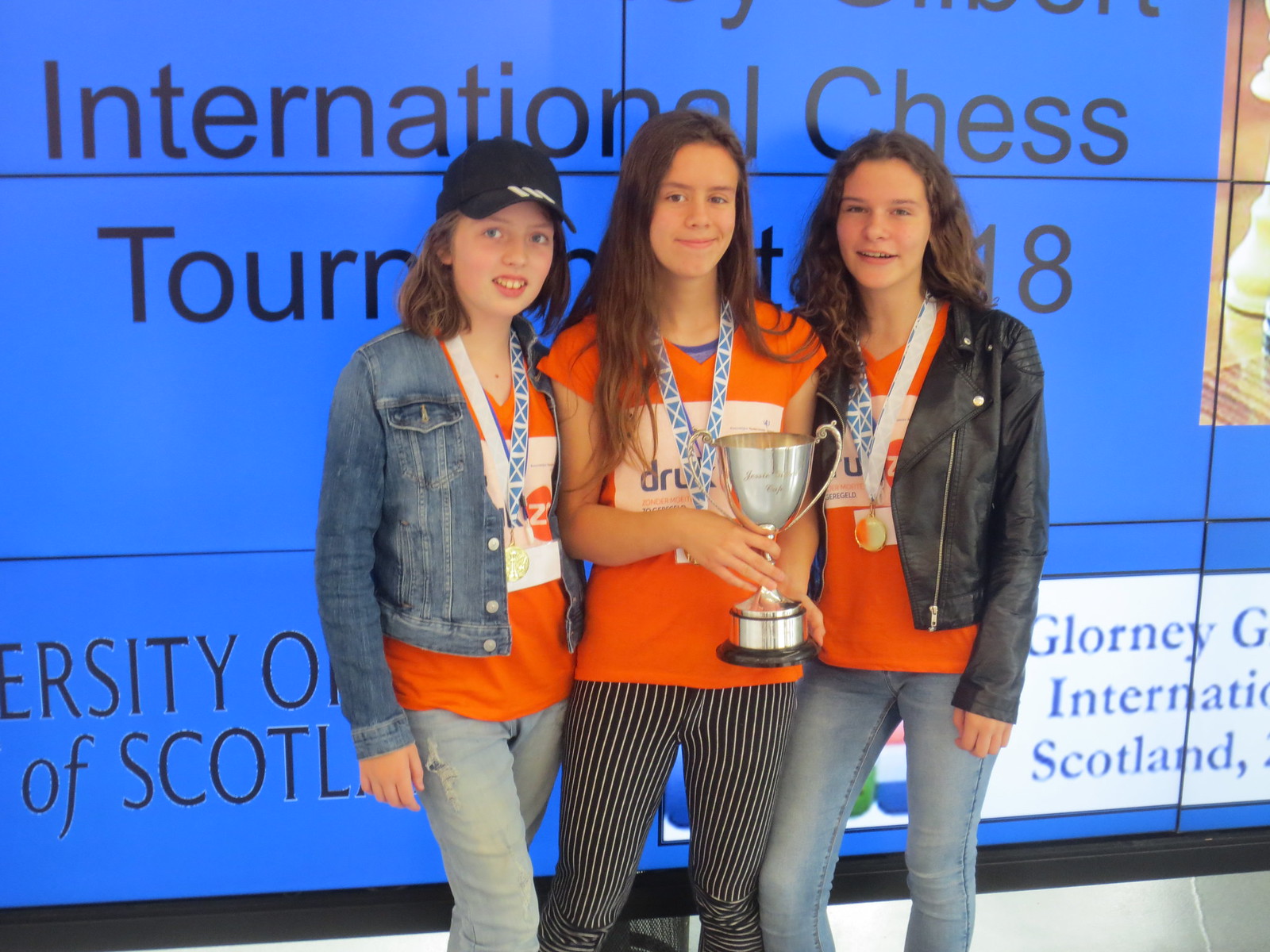The photograph showcases three teenage girls, likely between the ages of 12 and 15, standing shoulder to shoulder and smiling slightly. Each girl sports long brown hair and wears an orange t-shirt adorned with a white logo and a blue and white name tag necklace. The girl on the left completes her outfit with a black baseball cap, a denim jacket, and denim jeans. She also wears a name tag necklace. The middle girl pairs her orange t-shirt with black and white striped pants and proudly holds a small silver championship cup, resembling a miniature trophy one might win at a sports tournament. The girl on the right dons a black leather jacket over her orange t-shirt and wears denim jeans. All three girls display gold medals hanging from bands decorated with the Scottish flag. They stand against a blue wall with grid lines, which bears the words "International Chess Tournament" along with partially visible lettering that includes "University of Scottsdale" on the bottom left. The overall color palette of the image features blue, black, gold, silver, bronze, green, red, and white.